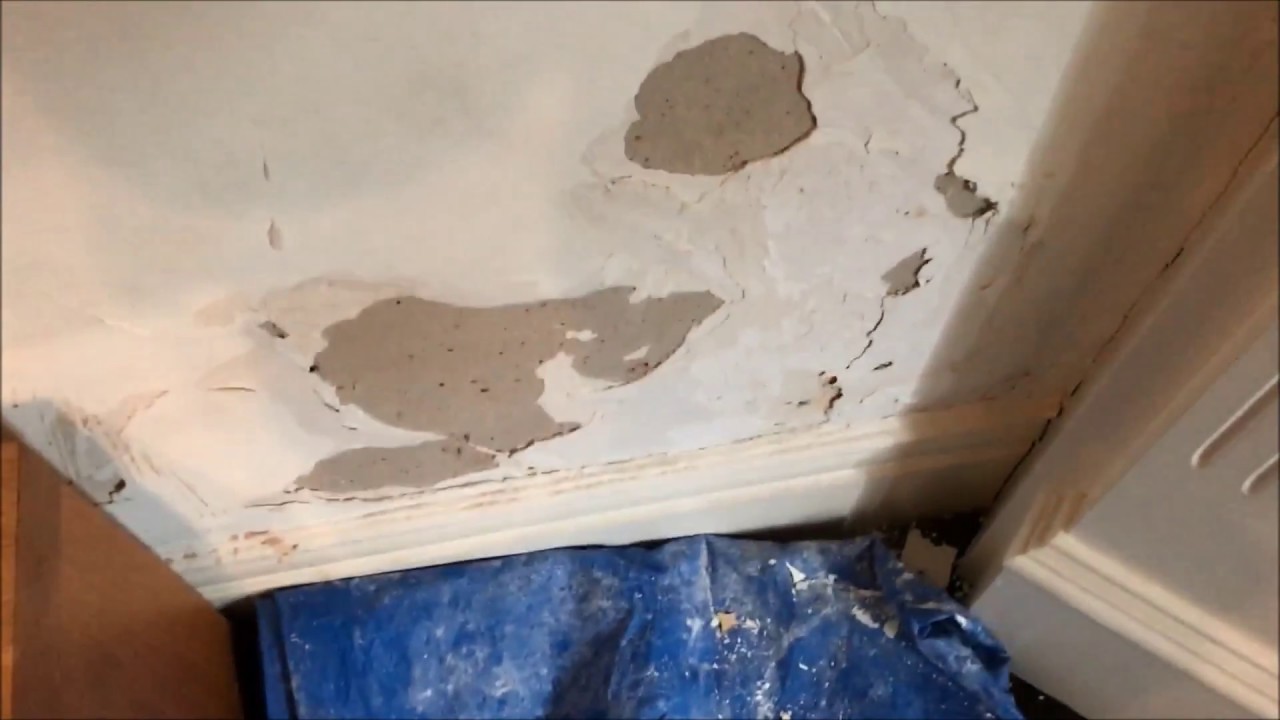This is a horizontal color photograph depicting a damaged white plaster wall on a house. The white paint on the wall is chipping and peeling off, revealing brown patches of the underlying material. The most prominent damage features a large circular area of exposed brown plaster, along with smaller sections of peeled-off paint near the lower portion of the wall. The white paint appears to be flaking off extensively, some of which has gathered on a blue tarp spread out at the bottom of the wall. The tarp itself is stained with white powder from the chipped paint. To the right side of the photograph, the wall transitions into a corner that extends diagonally out of the picture. On the left side, there is a brown object that descends to the lower left corner of the frame. It appears that someone has begun scraping the wall in preparation for repairs, evidenced by the scattering of paint flakes on the blue tarp and the visible cement behind the peeling paint. The wall also features a baseboard, adding to the structure's architectural detail.